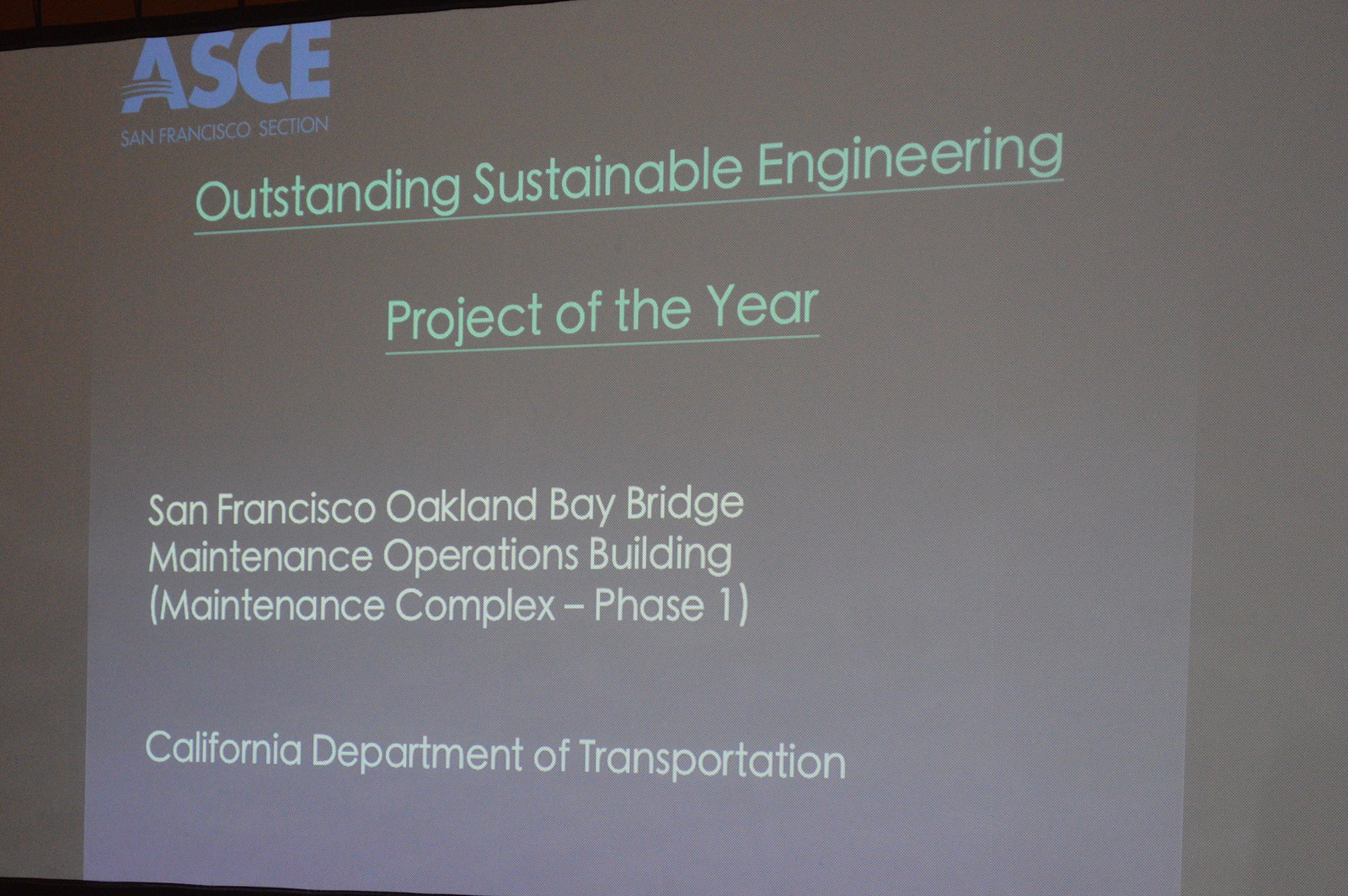This rectangular photograph captures a slightly angled view of a PowerPoint presentation slide projected onto a screen or white wall. At the top left corner, a blue logo reads "ASCE" with "San Francisco Section" in smaller font below it. Dominating the center of the slide, an underlined title in mint green announces the "Outstanding Sustainable Engineering Project of the Year." Directly beneath this title, in white text, the caption lists the "San Francisco-Oakland Bay Bridge Maintenance Operations Building" with the addition "Maintenance Complex-Phase 1" in brackets. At the very bottom of the slide, it credits the "California Department of Transportation." The slide background is primarily white or grayish, and there are small black triangles visible at the top and bottom left corners of the photograph. Various colored fonts and a distinct layout make the details of the text stand out against the slide's background.